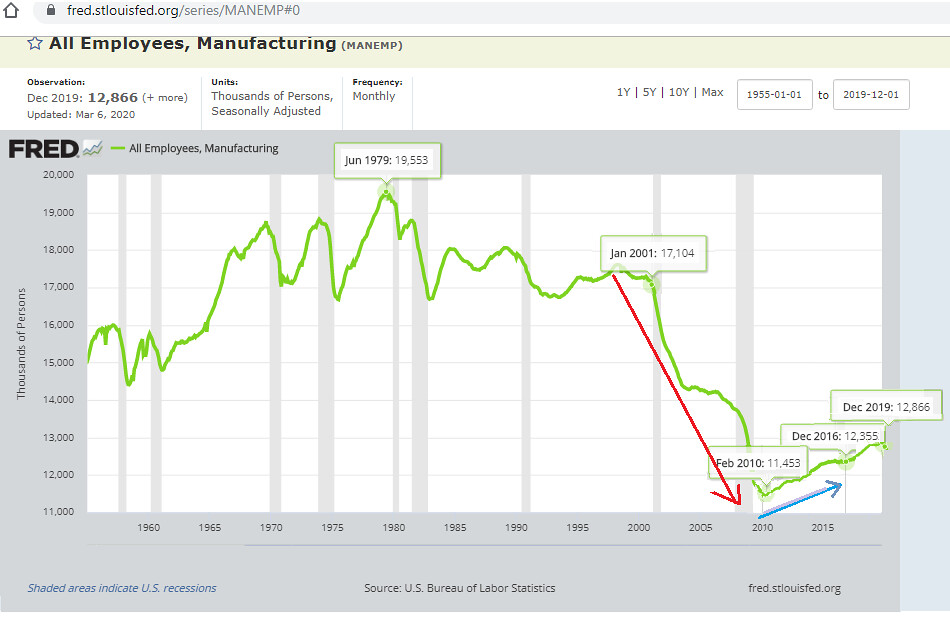This screenshot from a webpage (fred.stlouisfed.org/series/MANEMP#0) displays a detailed line graph labeled "All Employees: Manufacturing (MANEMP)." The chart's y-axis measures employment in thousands of persons, ranging from 11,000 to 20,000, while the x-axis spans from approximately 1955 to 2019. The data points are connected by a neon or lime green line, showing employment trends over time. Employment starts around 15,000 in the late 1950s, peaks at 19,553 in June 1979, and then sharply declines from 17,104 in January 2001 to 11,453 in February 2010. A red arrow highlights this significant drop. Post-2010, the employment figures gradually increase, marked by a blue arrow, but they do not recover to previous levels, ending at 12,866 in December 2019. The chart has a gray background and a white plot area, with adjustments for observation periods, units (thousands of persons), and seasonal adjustments noted on the right side of the page.